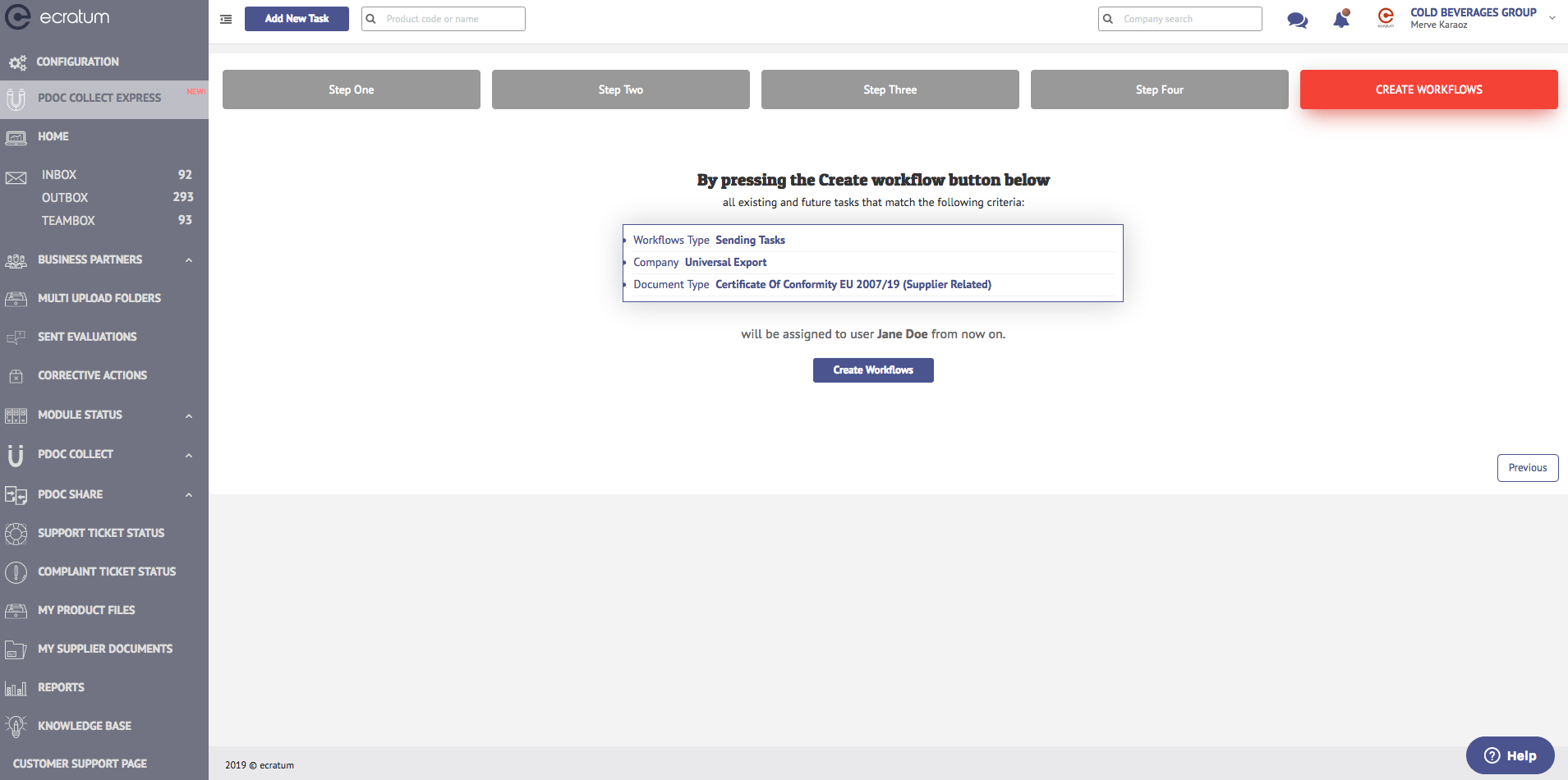Screenshot Description: The screenshot features a computer interface with a user-unfriendly design predominantly using grey as the background color and white text in a very thin font, making it difficult to read. A small black symbol is displayed at the top but does little to improve the visibility against the grey background. At the very top of the screenshot, there is a white bar featuring a blue button labeled "Add New Task," a search bar, and a series of icons, one of which leads to a section called "Cold Beverages Group."

In the left pane, there appears to be a vertical menu with a grey background, housing numerous options. Currently, an option labeled "Collect Express" is selected. Towards the right side of the interface, there are four steps listed vertically: step one, step two, step three, and step four. The step highlighted in red reads "Create Workflows." Below this, an instruction states, "By pressing the Create Workflow button below, it’s going to do so," indicating that the next action would be to create a new workflow. The interface seems to be preparing to assign tasks or workflows to users, although the cluttered and hard-to-read design obstructs effortless interaction.